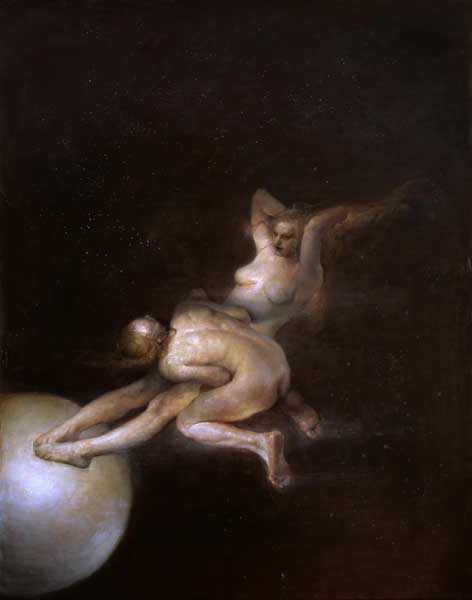In this detailed classical painting, set against a dark, almost black background, we see two human figures, both appearing nude. The composition is dominated by shades of brown and silvery gray. The first figure, a female, lies on her back with her hands behind her head, possibly grasping her hair. Her feet rest on a silvery brown sphere positioned in the lower left corner of the canvas, reminiscent of a modern exercise ball.

The second figure, which appears to be female partly due to the long hair, is kneeling just above the first figure’s midsection, facing left and bent over. This figure's back is towards the viewer, obscuring any view of the first woman's body below the knees and above the breasts. The pose of the kneeling figure’s arms, tucked below the abdomen, adds a layer of ambiguity.

Both figures’ nudity and their intertwined poses give the scene an almost ethereal and intimate, possibly even symbolic element, evoking interpretations of birth, interaction, or support. The striking contrast between the nude bodies and the dark void of the background enhances the painting's dramatic and mysterious atmosphere.